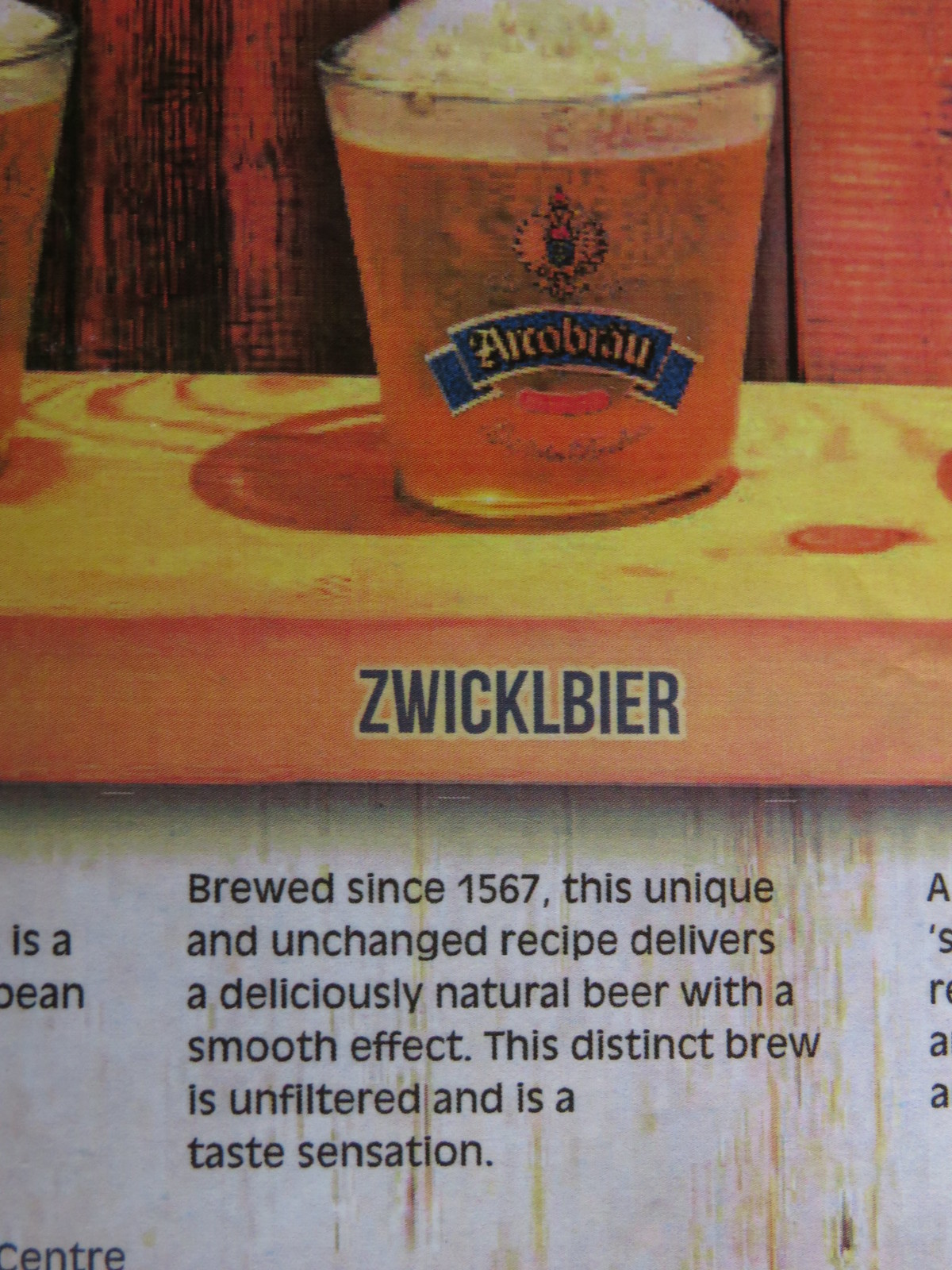This detailed close-up image features a glass of beer, showcasing its enticing foam head that crowns the top. The clear glass prominently displays a blue ribbon label with yellow lettering that reads "Arcobräu," topped with an insignia. The beer rests on a textured wooden plank, against which "Zwicklbier" is also displayed in blue text. Below the glass, a paragraph succinctly describes the beer: "Brewed since 1567, this unique and unchanged recipe delivers a deliciously natural beer with a smooth effect. This distinct brew is unfiltered and is a taste sensation." The rustic wooden surface adds a warm, inviting touch, making the beer appear even more appealing.